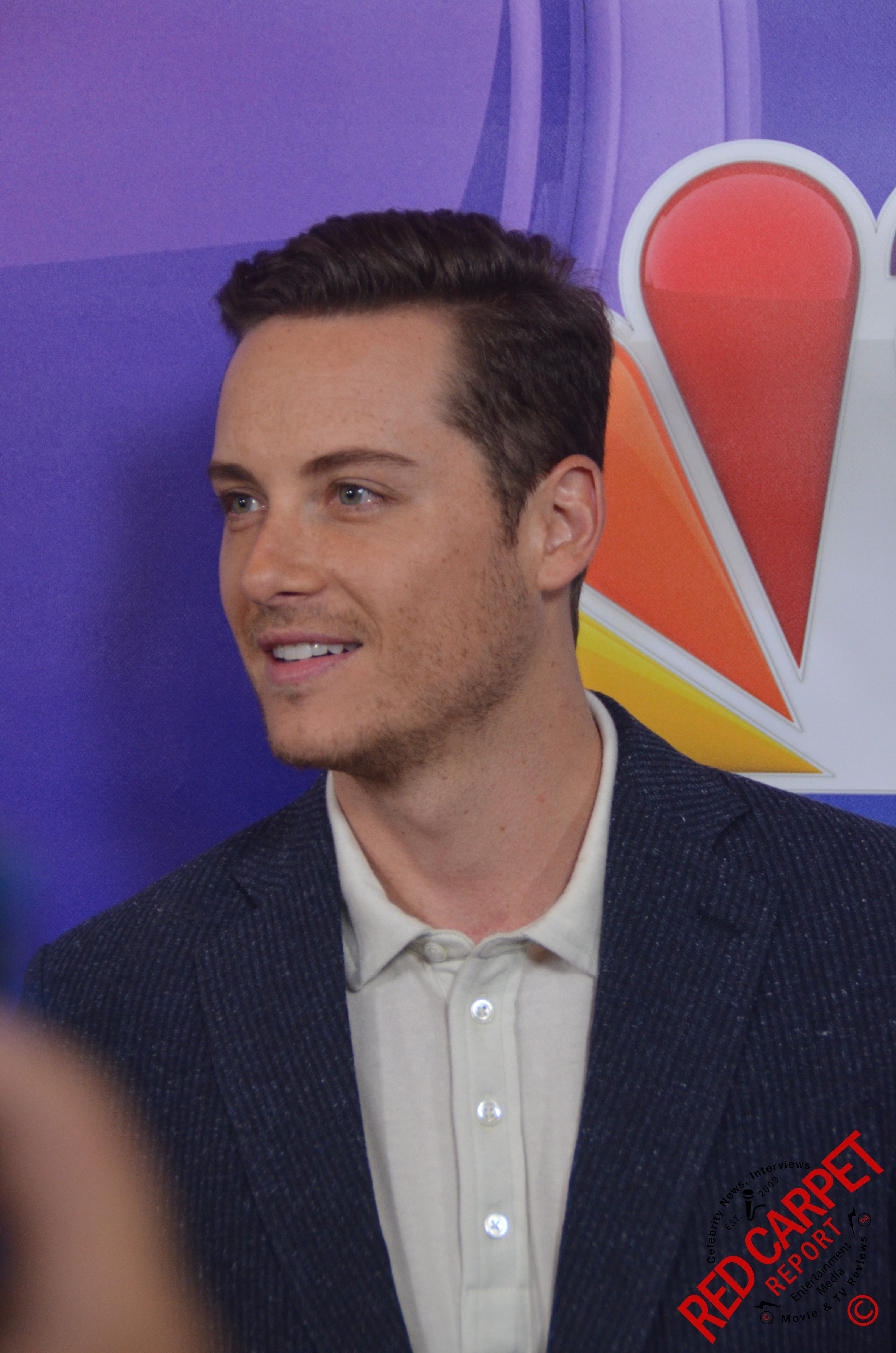In this image, we see a young man standing indoors, seemingly at an event. He is positioned directly in the center of the frame and is looking off to the left with a slight, open-mouthed smile. The man has short hair, parted to the left, and some stubble on his face. He is dressed in a dark gray or blue pinstriped suit jacket over a white or cream-colored button-down shirt, which resembles a polo shirt with the top button left undone.

The background of the image features a textured surface, possibly resembling robust paper or cardboard, predominantly in shades of purple. Off to the right-hand side of the image, slightly above the man’s shoulder, there is a colorful logo that closely resembles the NBC peacock symbol. This logo consists of several teardrop-shaped elements in different colors, specifically yellow, orange, green, red, and blue, converging at a single point.

In the bottom right corner of the image, there is text that reads "Red Carpet Report" written diagonally from left to right, with a copyright symbol beneath it. The overall color palette of the image includes various shades of purple, white, red, orange, yellow, tan, black, and gray. Additionally, there appears to be a blurry object, possibly someone’s finger, in the lower left corner of the photograph.